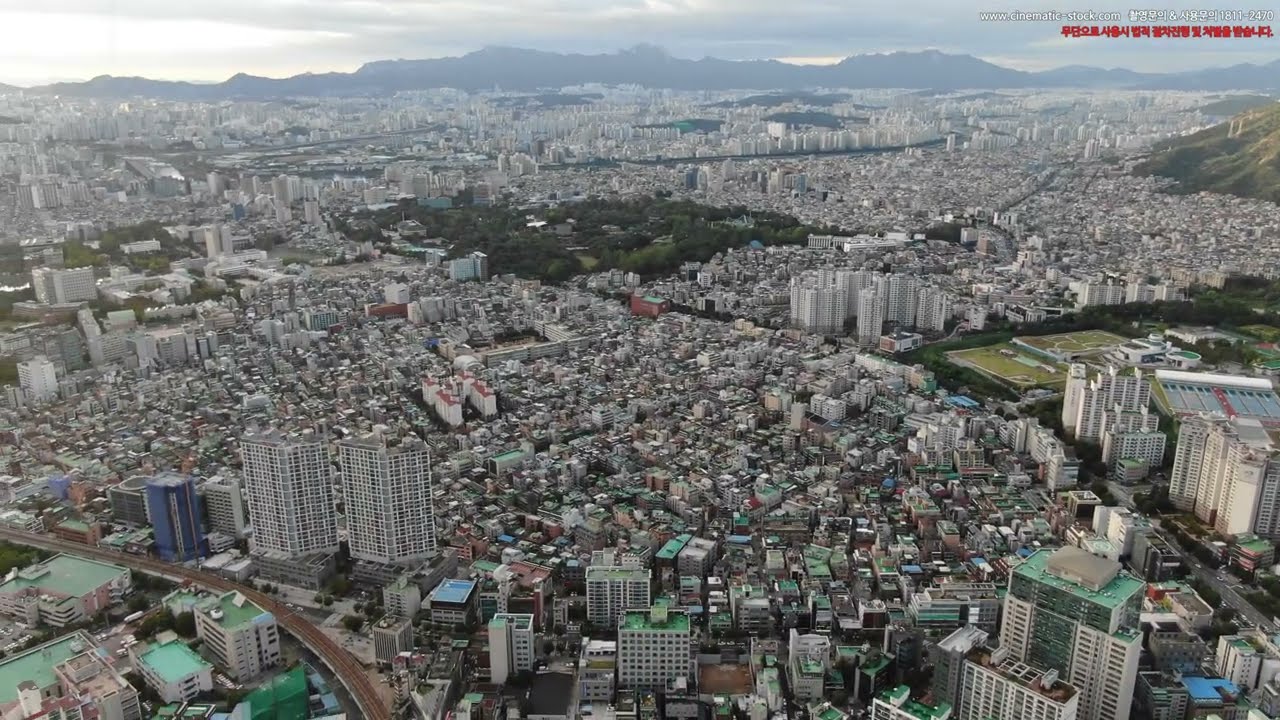This digital photograph captures a sprawling, densely populated metropolis from a high, elevated vantage point, likely taken from an airplane during the daytime. The city below is composed predominantly of multi-story, white buildings, many of which are topped with green rooftops, with some sporting blue roofs. In the lower left corner of the image, there is a brown street that curves to the left and is lined with buildings capped by mint green rooftops.

A large, grassy area reminiscent of Central Park can be seen towards the center of the city, providing a green contrast amidst the urban landscape. The background, occupying the top eighth of the image, features a thin row of mountains under a very dark, overcast sky, suggesting impending rain. The right side of the image also hints at additional grassy spaces, possibly fields or parks.

In the upper right-hand corner, there is a watermark that reads "www.cinematic-stock.com" followed by Asian lettering and the numbers "1811-2470." Below this, in red, are more Asian characters, adding to the likely Asian setting of the city. The overall color palette of the image includes white, green, blue, and shades of gray and black from the overcast skies.